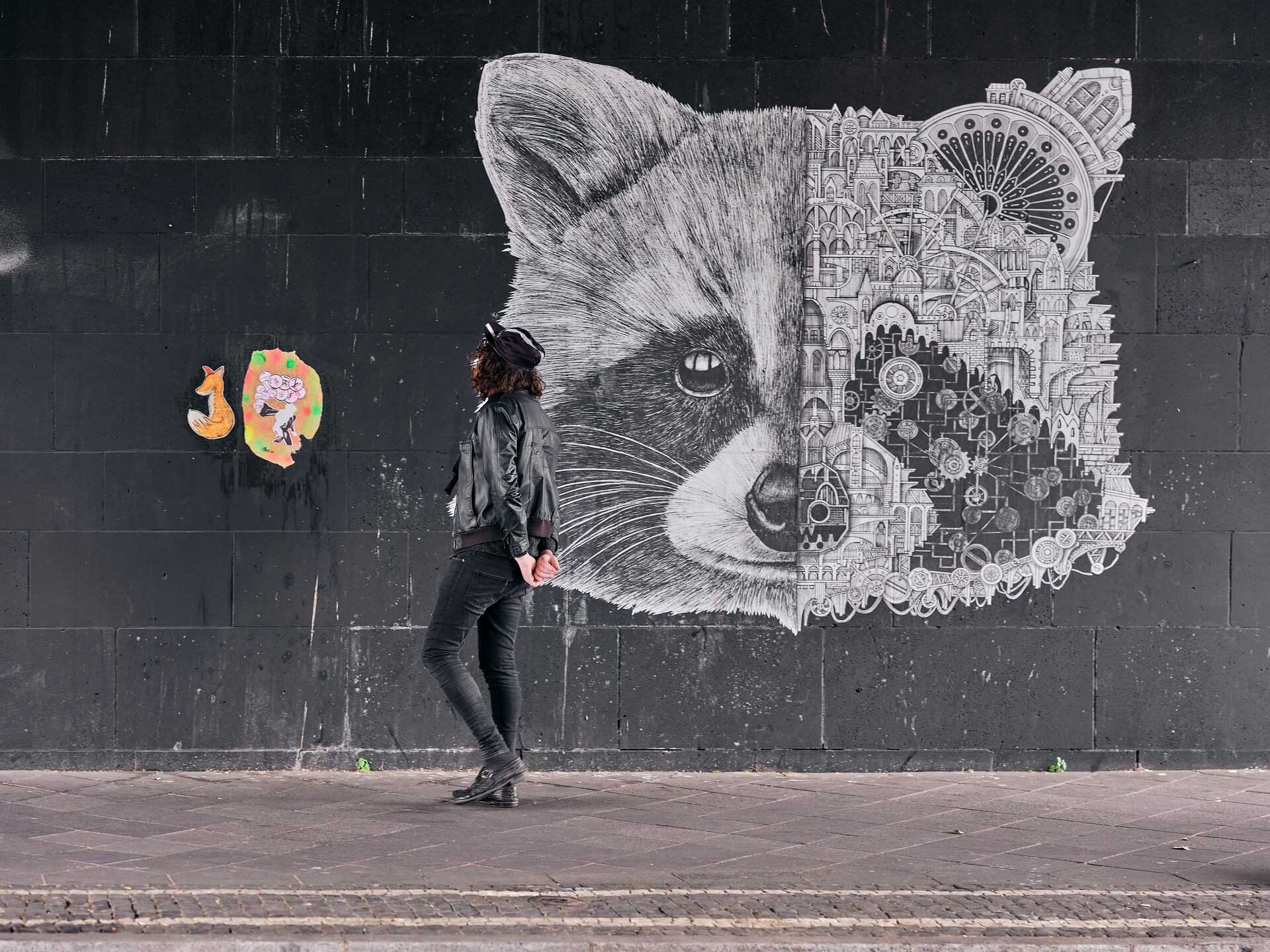The image captures a compelling street art scene with a meticulously detailed mural on a large, dark gray brick wall. The mural dominates the upper right quadrant of the wall and portrays a raccoon's face divided vertically. The left side of the raccoon appears lifelike with its characteristic black eyes and fuzzy fur, while the right side unveils an intricate steampunk interior composed of gears, wires, motors, and miniature cityscapes, all rendered in black and white.

In front of the mural stands a woman dressed entirely in black—donning a leather jacket, black jeans, black shoes, and a black hat. She is slightly off-center to the left and appears to be admiring a smaller, vividly colored piece of street art adjacent to the large mural. This smaller piece, located to her left, features an orange and green fox-like design, though its details are less perceptible. The ground beneath her consists of solid concrete squares, enhancing the urban aesthetic of the scene. Despite the absence of a visible artist's signature, the photograph highlights the impressive detail and creative composition of the street art.